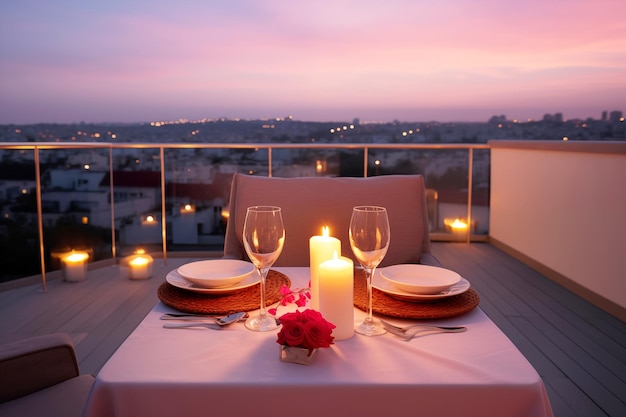The image depicts a romantic rooftop dinner scene set atop a building, bathed in the soft hues of a sunset. The table is elegantly arranged with a light pink tablecloth, adorned with a square glass bowl holding rose heads, and scattered rose petals. There are two white plates, each paired with round white bowls and set on circular woven placemats. Two wine glasses and lit candles also grace the table, casting a warm glow. Utensils including forks and knives are neatly placed, and beige chairs flank the table. Surrounding the setting, a glass barrier encloses the area, and additional candles can be seen on the ground. The sky transitions from purplish shades to a faint reddish-orange, reflecting the approaching twilight, while the city skyline with residential buildings is visible in the background. The entire scene exudes a feeling of intimate anticipation, waiting for guests to arrive.